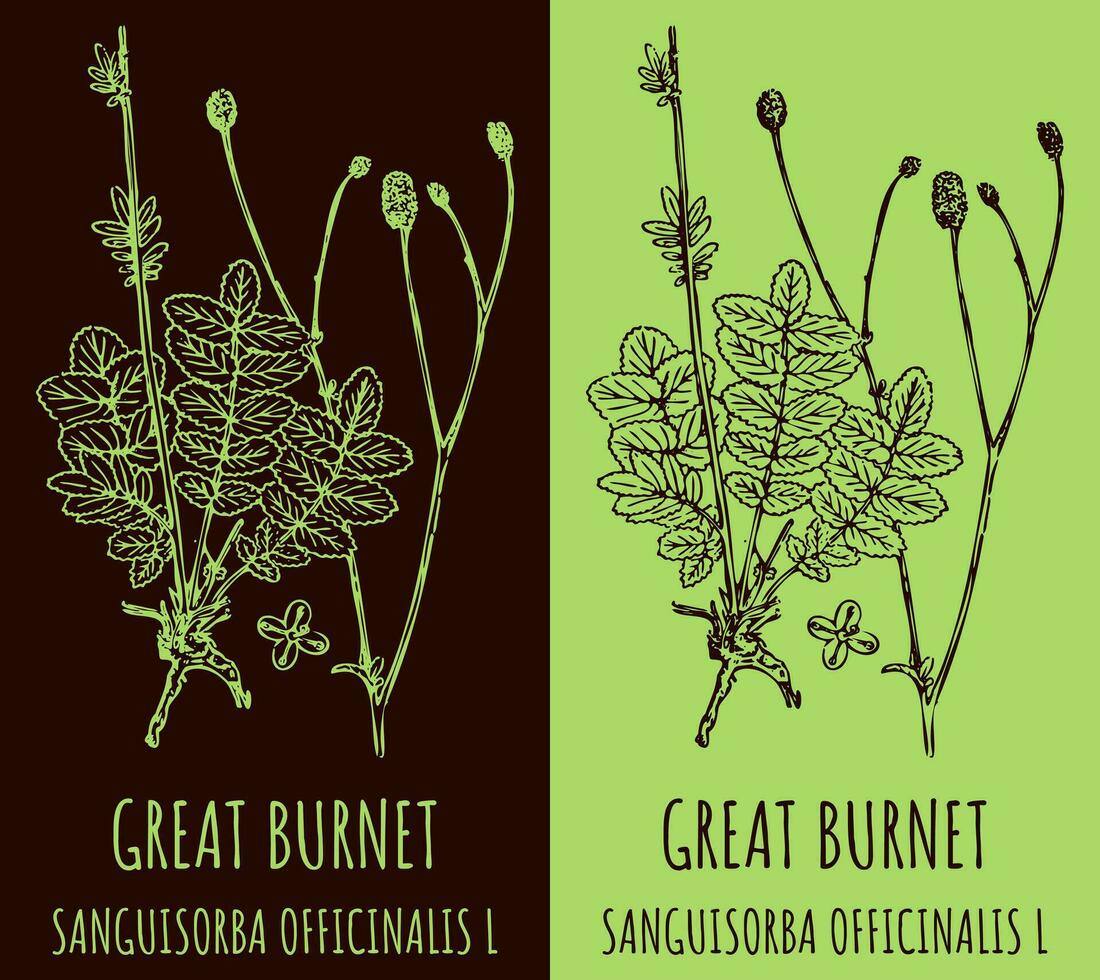In the hand-drawn image, two identical illustrations of plant leaves and branches are placed side by side, each showcasing an inverted color scheme. The left image features a dark brown background with light green leaves, labeled "Great Burnet" with its scientific name "Sanguisorba officinalis L." in green text beneath. The right image mirrors this composition but swaps the colors: it has a light green background with the plant details and text in a darker, almost black tone. This detailed artwork, reminiscent of botanical illustrations found in plant identification books, highlights the elegant structure of the Great Burnet plant through its contrasting color palettes.